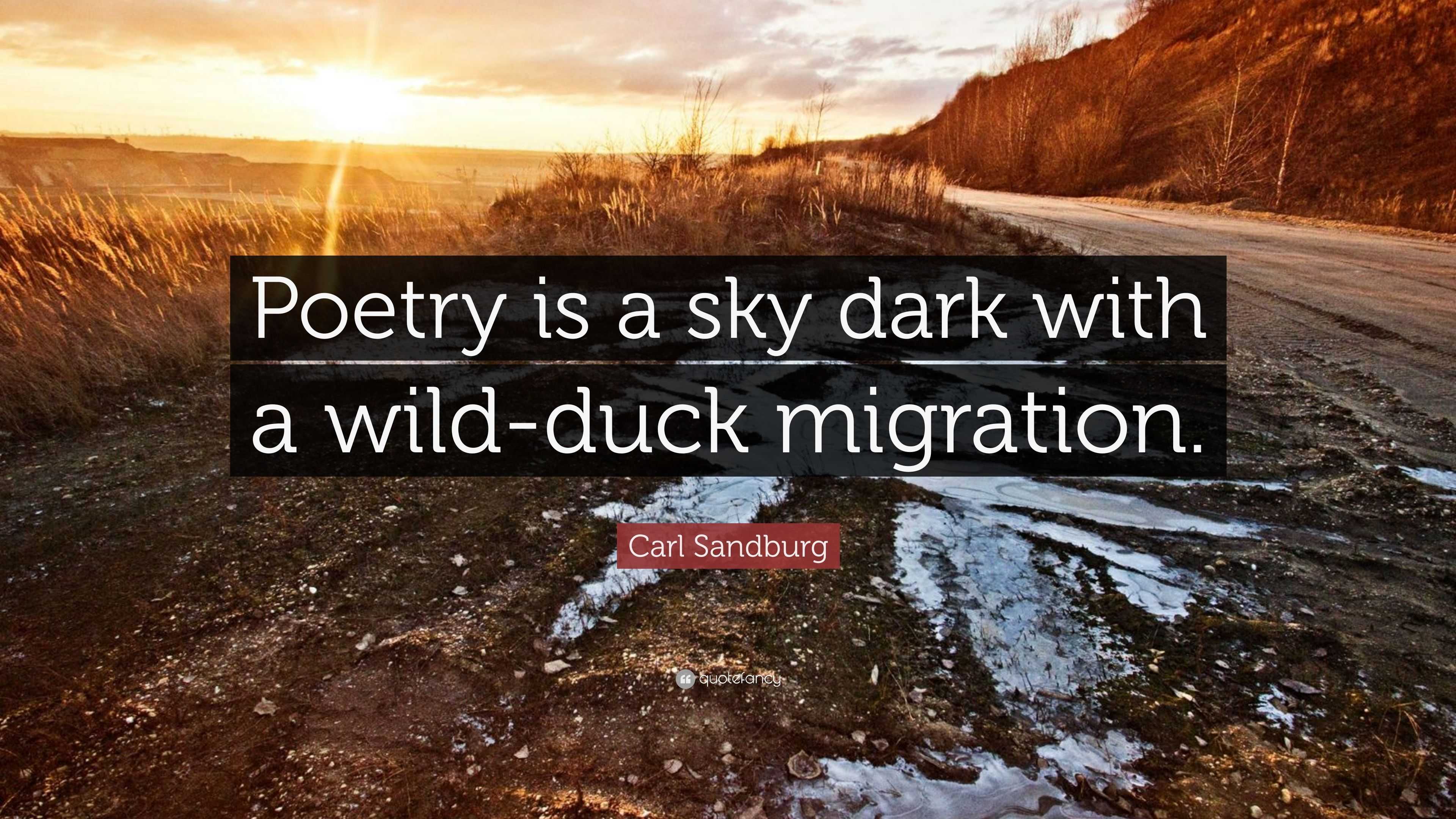The horizontal image portrays a rugged, late fall or early spring scene that appears to be set in the Western United States. A dirt road dominates the foreground, lined with ruts possibly formed by tires, and traces of ice glint in the cool air. Surrounding the road, the landscape is marked by burned-out grasses and exposed dirt. The rising or setting sun peeks over the horizon, casting a golden hue across the predominantly brown and yellow terrain. To the right, gently sloping hills add depth to the scene, though their sparse vegetation remains tinged with the season's brown shades.

At the center of the image, a striking quote is displayed in bold, black blocks with white text: "Poetry is a sky dark with a wild duck migration." Beneath this, in smaller white text on a red banner, the name Carl Sandburg is prominently featured. Tiny, unreadable white text appears just below the quote, adding a subtle detail to the overall composition. The image evokes a sense of solitude and reflective beauty, typical of the kinds of evocative quote-centric photos often found on inspirational sites.